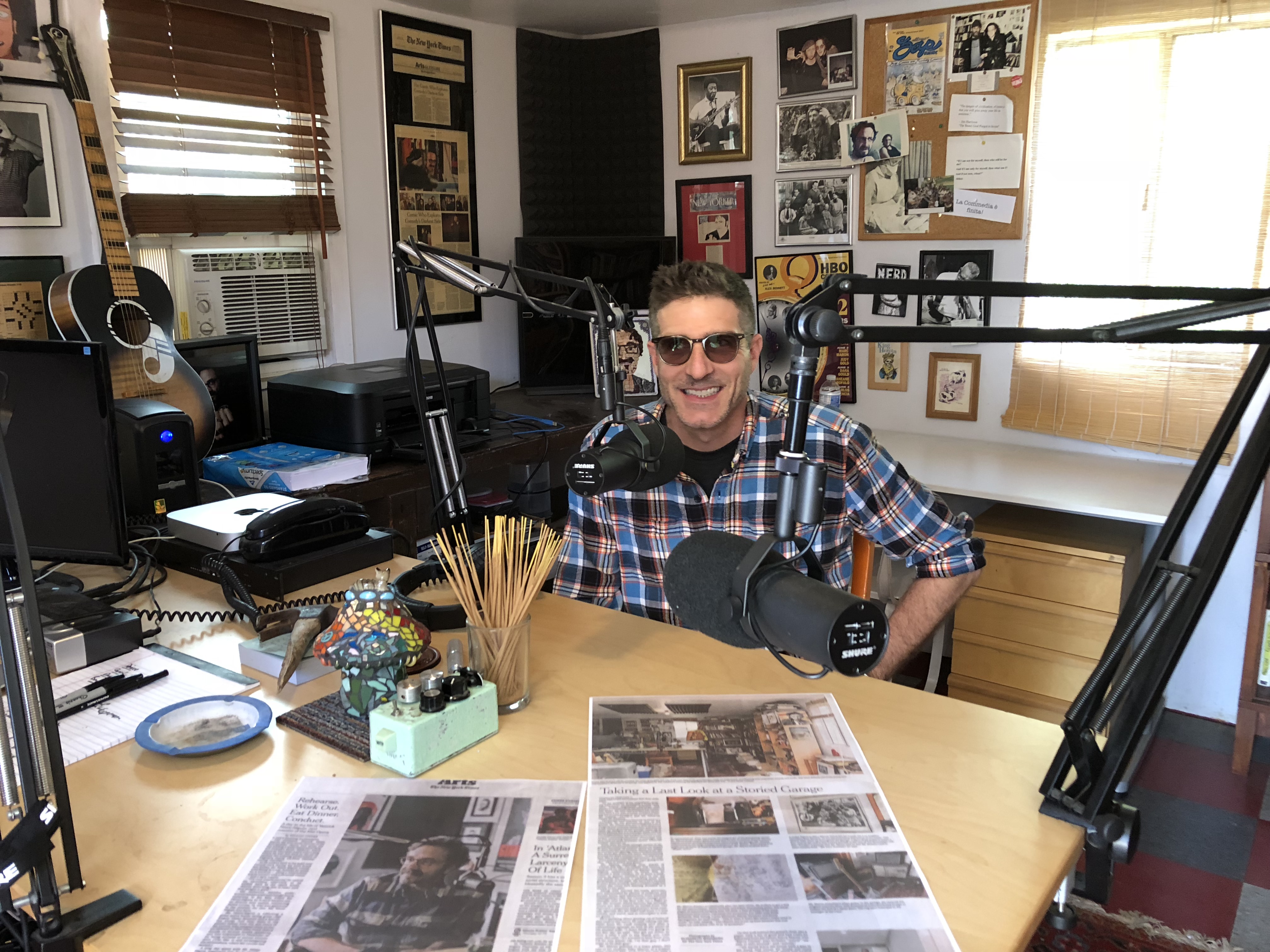The photograph, taken in a home studio, displays a man with short spiked dark hair wearing brown sunglasses and a blue checkered shirt, smiling at the camera. He is seated behind a small, thin wooden table cluttered with newspapers, a jar of straws, and various other items. Two large microphones, attached to adjustable metal poles, are pointed at him. The scene is complemented by a guitar propped up against the far wall. The walls of the room are adorned with numerous posters and pictures of celebrities and musicians, adding a vibrant touch to the space. The studio also features essential office equipment, including computers, printers, telephones, and bundles of A4 sheets, creating a busy yet organized atmosphere. Additionally, the room has windows on both walls, one of which houses an air conditioning unit, its blinds drawn to let in natural light.